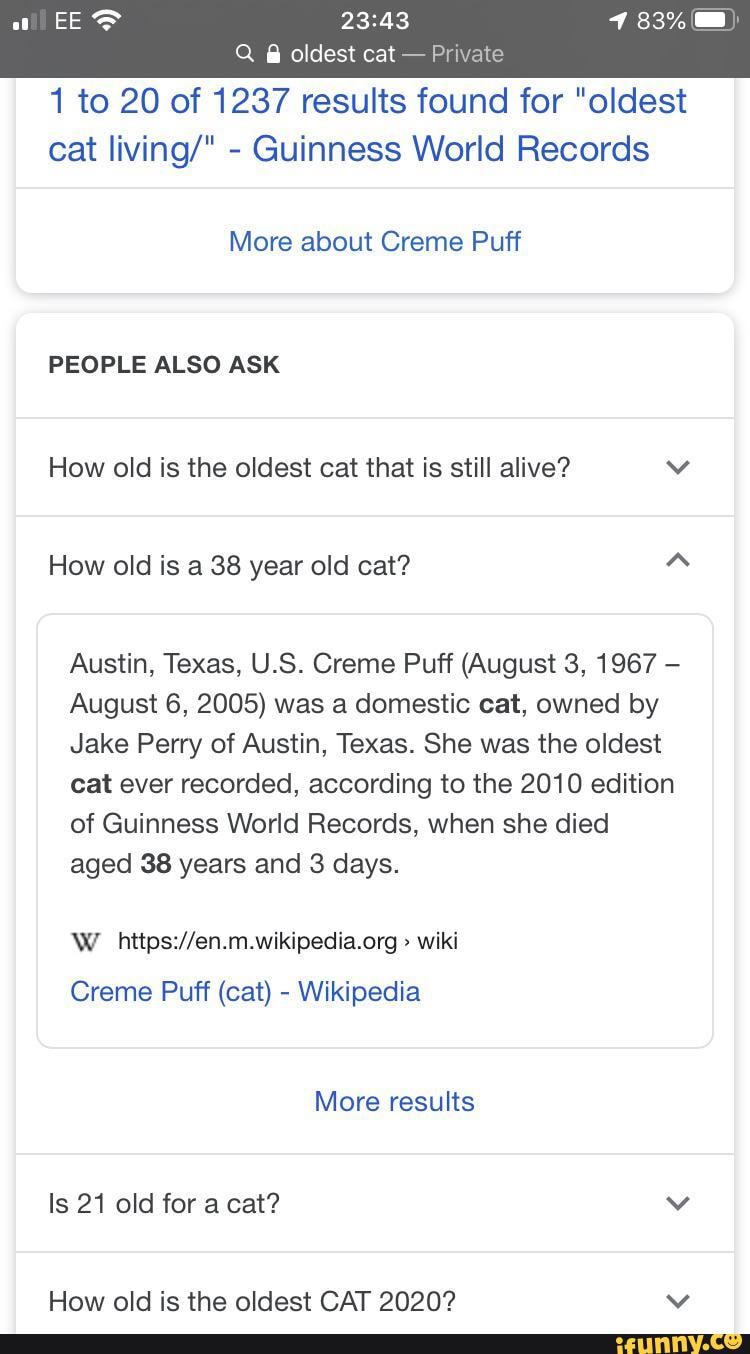A screenshot of a phone screen displays a search query entered using military time "2343" (11:43 PM). The search results headline reads "1 to 20 of 1,237 results found for oldest cat living in Guinness World Records." One prominent result discusses "Cream Puff," who holds the record for the oldest cat ever recorded. Cream Puff was a domestic cat born on August 3, 1967, and lived until August 6, 2005, reaching an age of 38 years and three days. She was owned by Jake Perry in Austin, Texas. This information is corroborated by both Guinness World Records and Wikipedia, where a link labeled "Cream Puff (cat)" and Wikipedia in blue text is displayed. The search also reveals related questions such as "How old is the oldest cat that is still alive?" and "How old is a 38-year-old cat?" Additional results explore topics like "Is 21 old for a cat?" and search variations for the oldest cat as of 2020. The screenshot comprehensively documents the search for record-holding cats, highlighting Cream Puff's notable longevity.